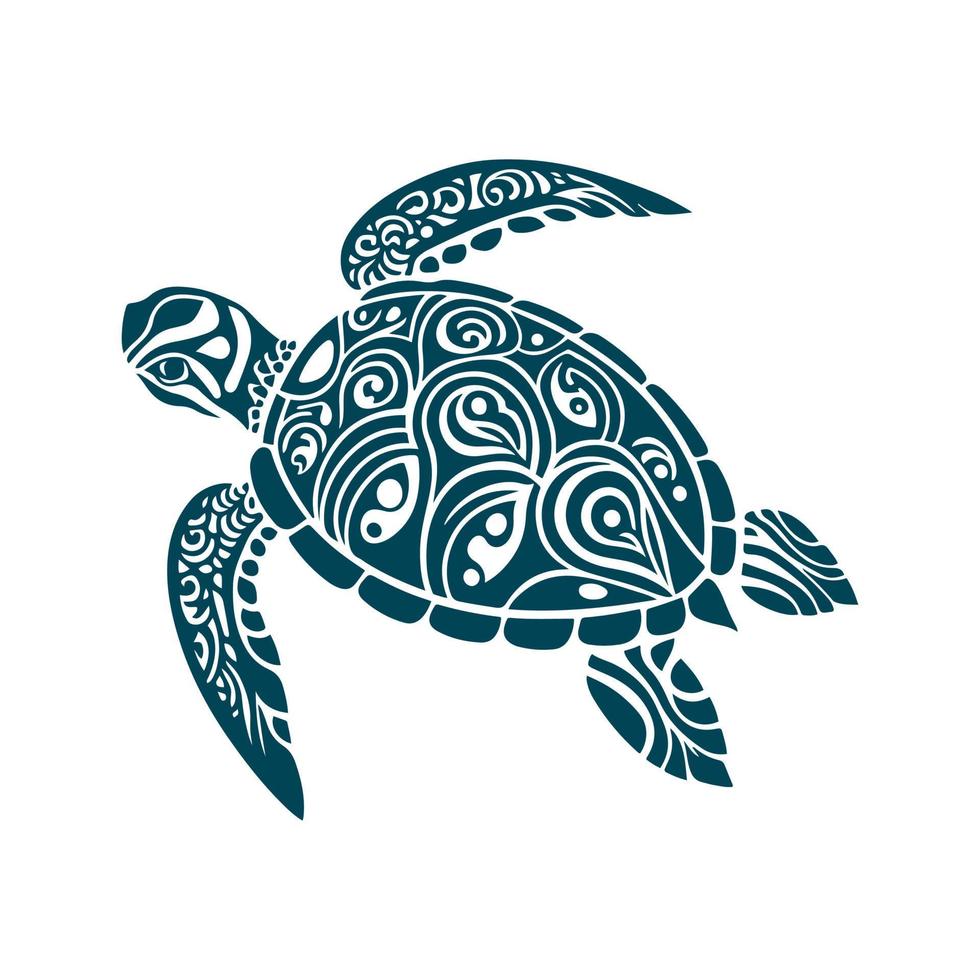The image is a detailed illustration of a sea turtle, positioned at a 45-degree angle, swimming upwards and to the left. Rendered in a striking mix of teal-green and blue ink, the design uses the white background to emphasize the intricate flowery and swirling patterns adorning the turtle's shell and flippers, reminiscent of Hawaiian or Pacific Islander art. The sea turtle's front flippers extend out like wings, while its rear flippers trail behind. Only one eye is visible, gazing towards the left, enhancing the sense of motion through an unseen current. The entire composition stands out against the stark white backdrop, focusing all attention on the elaborate and vibrant design of the sea turtle itself.